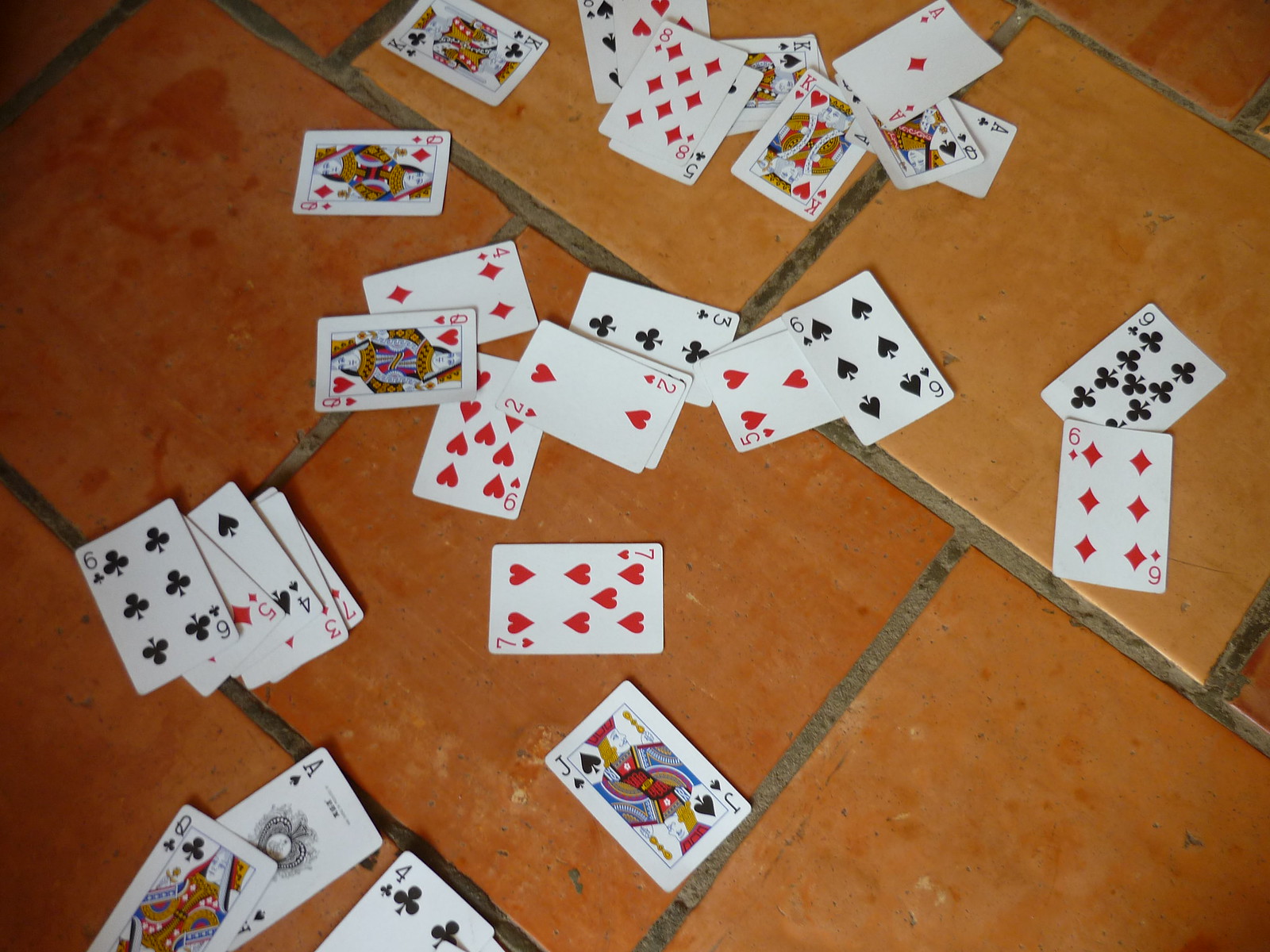A close-up image depicts a scattered deck of playing cards spread haphazardly across a tiled floor. The floor is composed of large square tiles in varying shades of golden brown and orange, creating a vibrant and warm backdrop. The cards lie face-up in a random arrangement, displaying a mix of suits: spades, hearts, diamonds, and clubs. Notably, a joker card is positioned toward the lower section of the image, while an ace card is also visible. In the lower left corner, a queen of clubs stands out with its distinctive black club symbol. Additionally, among the assortment, the six of diamonds and the six of spades can be clearly identified.